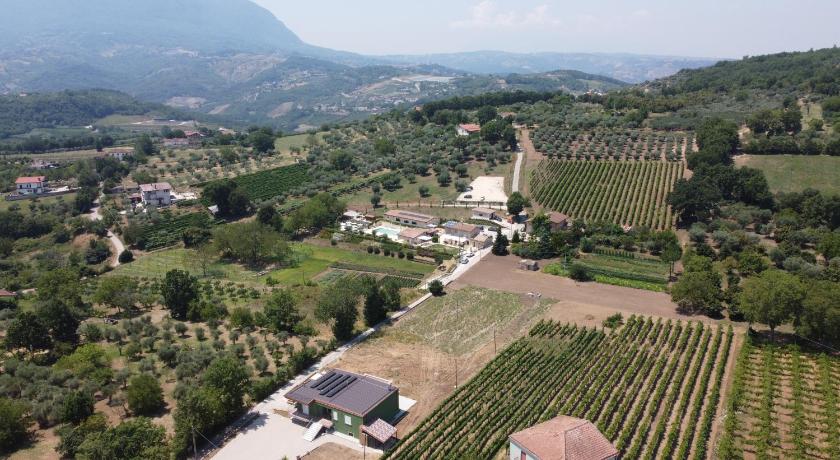This is an aerial view of a picturesque countryside captured from an elevated angle. The vast expanse of land is sectioned into numerous rectangular fields, meticulously organized with rows of green crops. Here and there, clusters of newly planted trees break the uniformity of the fields. Scattered throughout are several individual houses, adding a human touch to this predominantly agricultural landscape. A road weaves through the middle of the image, flanked by trees and fields, and it vanishes into the distance on the right side. In the backdrop, majestic, undulating hills and mountains frame the scene, draped in a light blue sky adorned with sporadic clouds. The bottom segment of the image features open grassland interspersed with rows of trees and additional fields, offering a glimpse of the region's natural beauty and agricultural bounty.